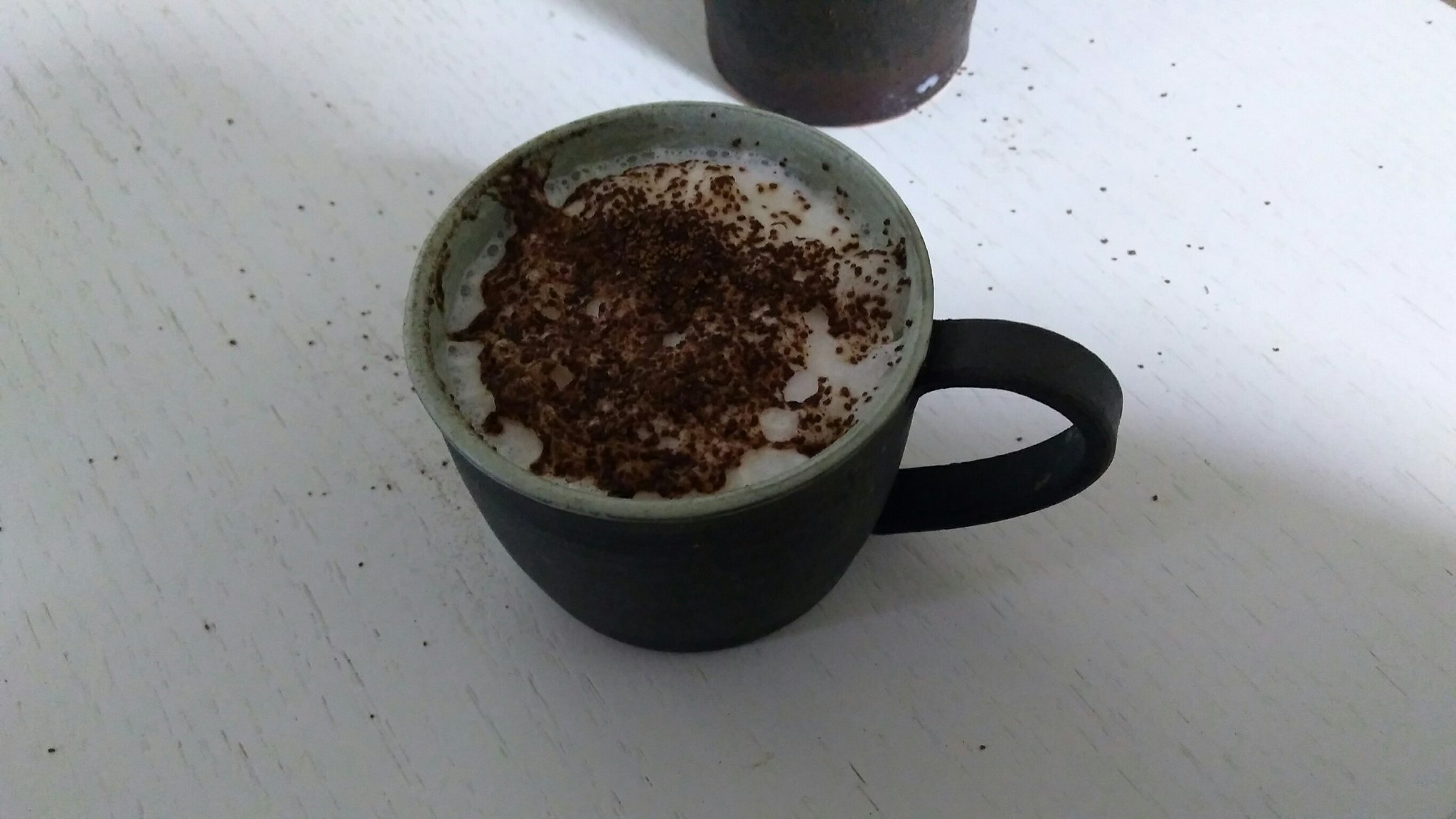This indoor photograph features a dimly lit scene focused on a single coffee cup placed centrally on a whitish, woodgrain-painted table. The cup appears to be a dark color, possibly black or dark cobalt blue, and has a lighter interior, perhaps light gray. The handle of the cup faces to the right. Inside the cup, there is a frothy, milky beverage topped with brown sprinkles, which could be chocolate, coffee grounds, or cinnamon. Additionally, the image captures the bottom portion of another dark-colored mug at the top of the frame, partially visible and slightly out of focus. The table around the cup is also speckled with a few of these brown sprinkles, adding texture to the scene. Overall, the photograph presents a cozy, intimate coffee moment, albeit with lighting that leaves some details difficult to discern.